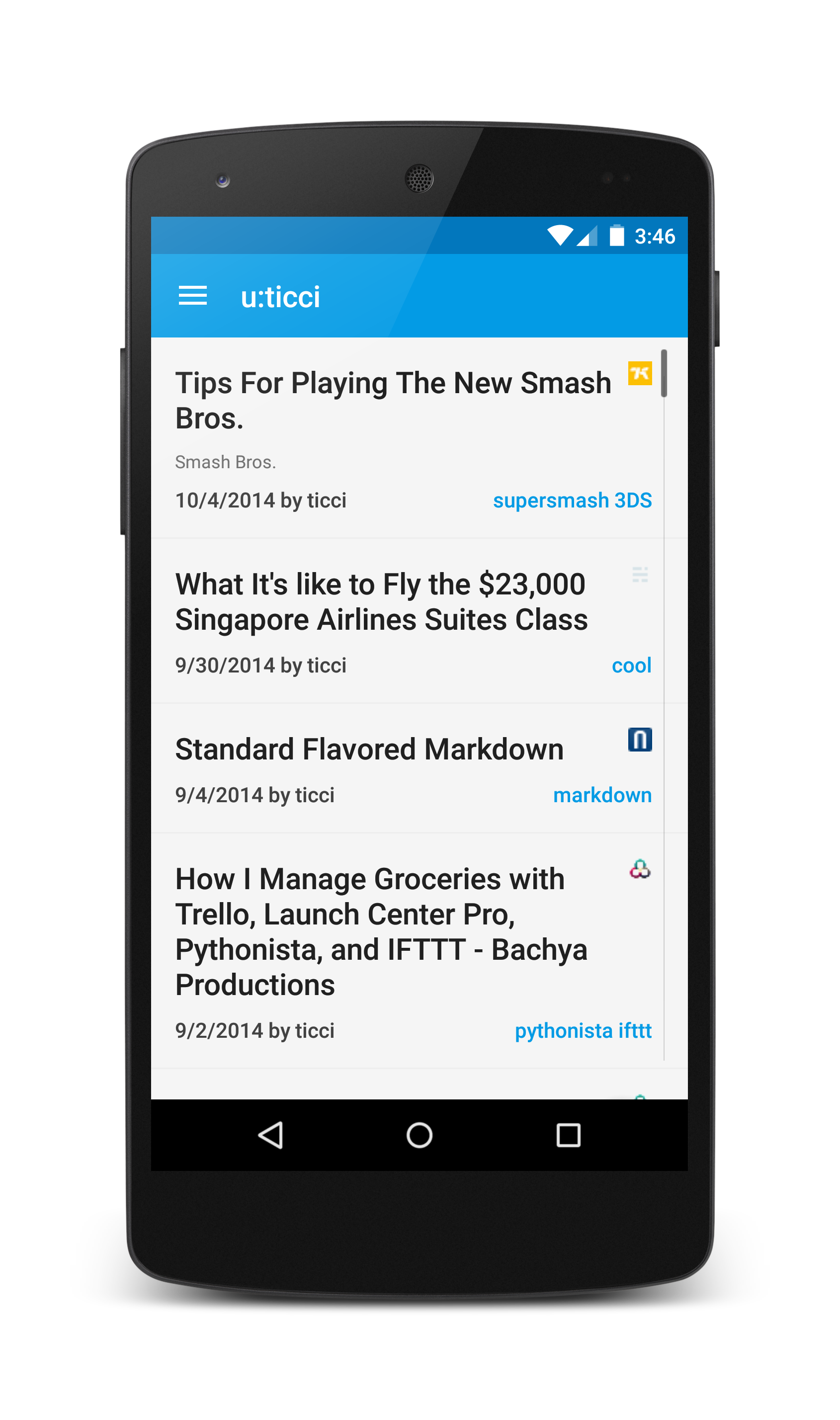The image features a close-up of a smartphone with a nearly black, dark gray case. On the right side of the phone, there is an on/off button, while the left side near the top has the volume controls. At the center top of the smartphone, a round indentation likely functioning as a speaker is visible.

The screen displays a user interface with a dark blue border at the top, which fades into a lighter blue at the bottom. The blue border contains the text "U:T-I-C-C-I." Below this border, the screen has a predominantly white background featuring various texts and information. The main content on the screen includes:

- "Tips for playing the new Smash Brothers, Smash Brothers 10/4/2014 by T-I-C-C-I, Super Smash 3DS."
- "What it's like to fly the $23,000 Singapore Airlines Suites Class, 9/30/2014 by T-I-C-C-I, cool."
- "Standard flavored markdown, 9/4/2014 by T-I-C-C-I markdown."
- "How I manage groceries with Trello, Launch Center Pro, Pythonista, and IFTTT - Batchia Productions, 9/2/2014 by T-I-C-C-I, Pythonista, IFTTT."

Text elements such as "Super Smash 3DS," "cool," "markdown," and "Pythonista, IFTTT" are highlighted in blue and aligned to the right side of the screen.